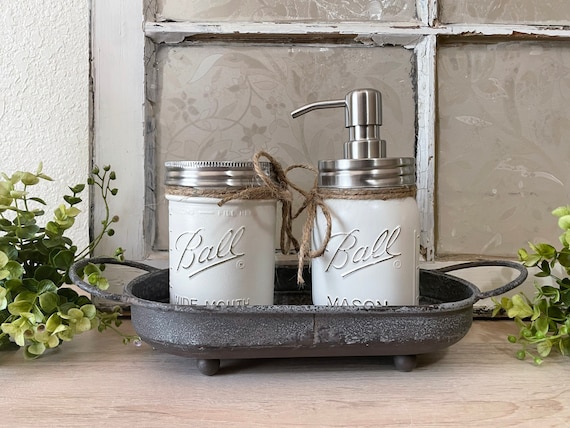This is a photograph depicting a rustic decor scene, possibly set in a kitchen or bathroom. Central to the image are two white-painted mason jars labeled "Ball," each adorned with a silver lid. One jar features a pump spout, likely used for dispensing soap, while the other has just a lid. These jars rest in a small, gray metal container with two side handles, designed with small ball feet. Surrounding the metal container are artificial green leaves, adding a touch of nature to the setup. The background reveals a window that is either painted over or covered with paper, preventing any view outside. The entire arrangement sits atop a wooden surface, further enhancing the cozy and homey atmosphere of the scene.